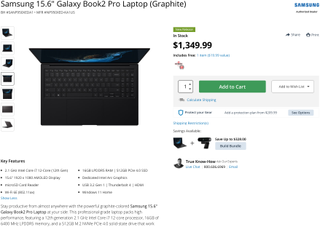A screenshot from presumably the Samsung website or another authorized retailer showcases the Samsung 15.6-inch Galaxy Book 2 Pro laptop in its sleek graphite color. The image lacks any retailer-specific URL or logo, but prominently displays the Samsung logo in bold blue text at the top right corner. Dominating the left-hand side is the product title: "Samsung 15.6-inch Galaxy Book 2 Pro Laptop Graphite," accompanied by a model and serial number.

Seven thumbnail images of the laptop in various angles and perspectives are aligned vertically on the left. The selected image of the moment is the fourth thumbnail, which offers an overhead view primarily focusing on the keyboard, with the screen slightly tilted.

On the right side of the screenshot, the product is marked as in stock, priced at $1,349.99. Below this, a quantity selector is situated next to a green "Add to Cart" button. Adjacent to this is a white button with gray text labeled "Add to Wishlist." Further down, there's a gentle prompt suggesting a bundle deal with another product, followed by a paragraph outlining the key features and specifications of the laptop.